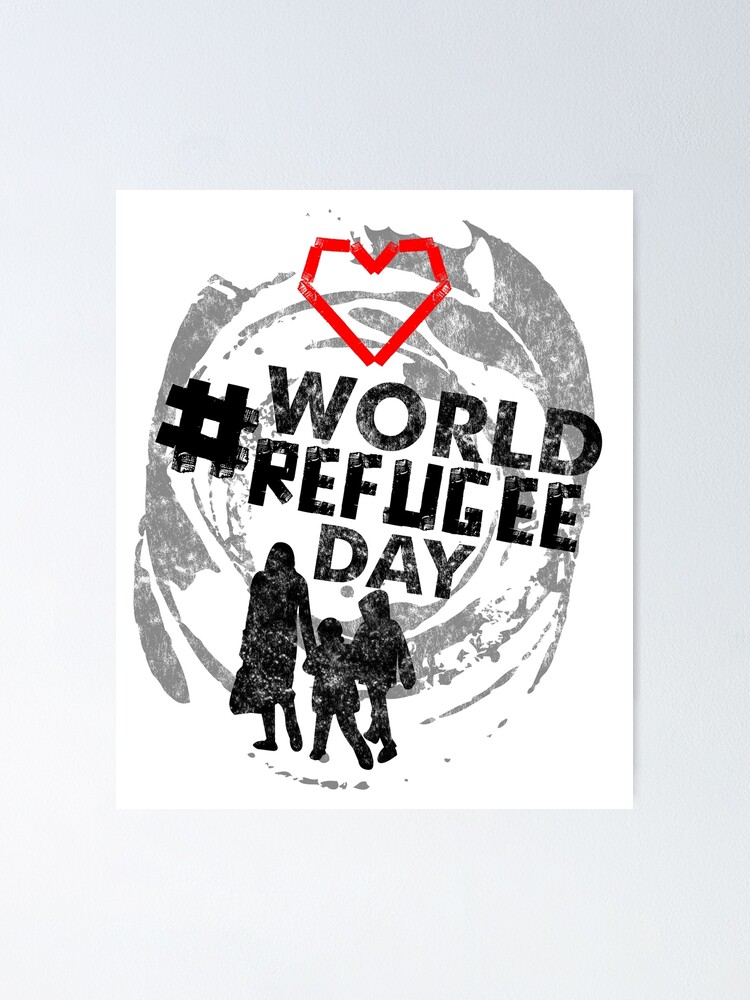The image is a vertical, rectangular information poster for World Refugee Day, set against a light gray background. At its center is a white flyer styled with a screen-printed effect. The design features a series of thin and wide black lines, spiraling inward from the edges towards the center, creating a dynamic yet subtle background. At the top of the flyer is a jagged red heart, positioned prominently above bold, capitalized text that reads "WORLD REFUGEE DAY." To the left of this text is a pound sign (#). Below the words, there is a shadowy silhouette of three people: a mother on the left holding a bag in her left hand and gripping the hand of a small child with her right. This child is also holding the hand of an older sibling on the far right. The entire composition combines black, white, and red hues to communicate a powerful message about the significance of the day.